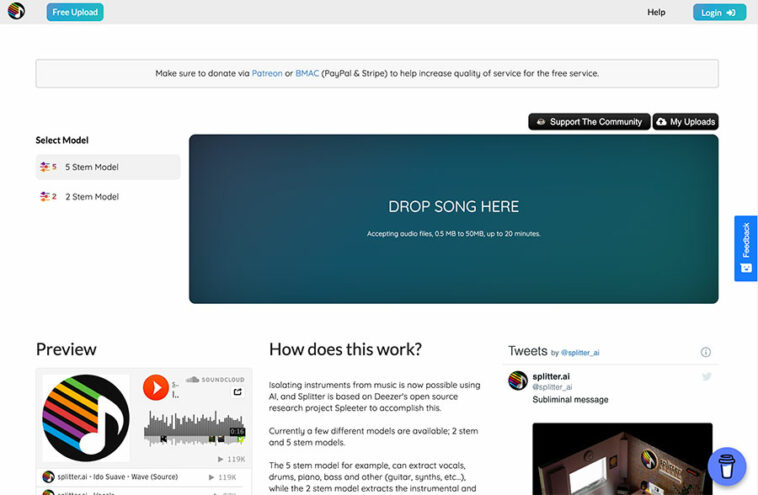A detailed caption for the described image could be:

---

This image showcases a web page dedicated to music uploading. In the upper left corner, a prominent blue button labeled "Pre-Upload" is visible. Across from it, in the upper right corner, there is another blue button labeled "Log In," with a simplistic black-text "Help" link situated just to its left.

Dominating the center of the page is a large, dark blue rectangular box with the text "Drop song here" prominently displayed. This area specifies that it accepts audio files between 0.5 megabyte and 50 megabyte, and allows for tracks up to 20 minutes in length. Above this central upload box, two black buttons labeled "Support the Community" and "My Uploads" are aligned horizontally.

Further up, a noticeable banner urges users to donate via Patreon or BMAC, PayPal, and Stripe to enhance the quality of this free service. Below the main upload section, there is a "Preview" button which enables users to play their uploaded music on SoundCloud, accompanied by a brief description of how the website operates, despite the small and challenging-to-read text. To the right, there is a mention of the Twitter page for this platform, identified as ’@splitter.ai’, along with the tagline "subliminal messages."

---

This caption provides a comprehensive and detailed description of the image, highlighting key elements and their positions on the web page.